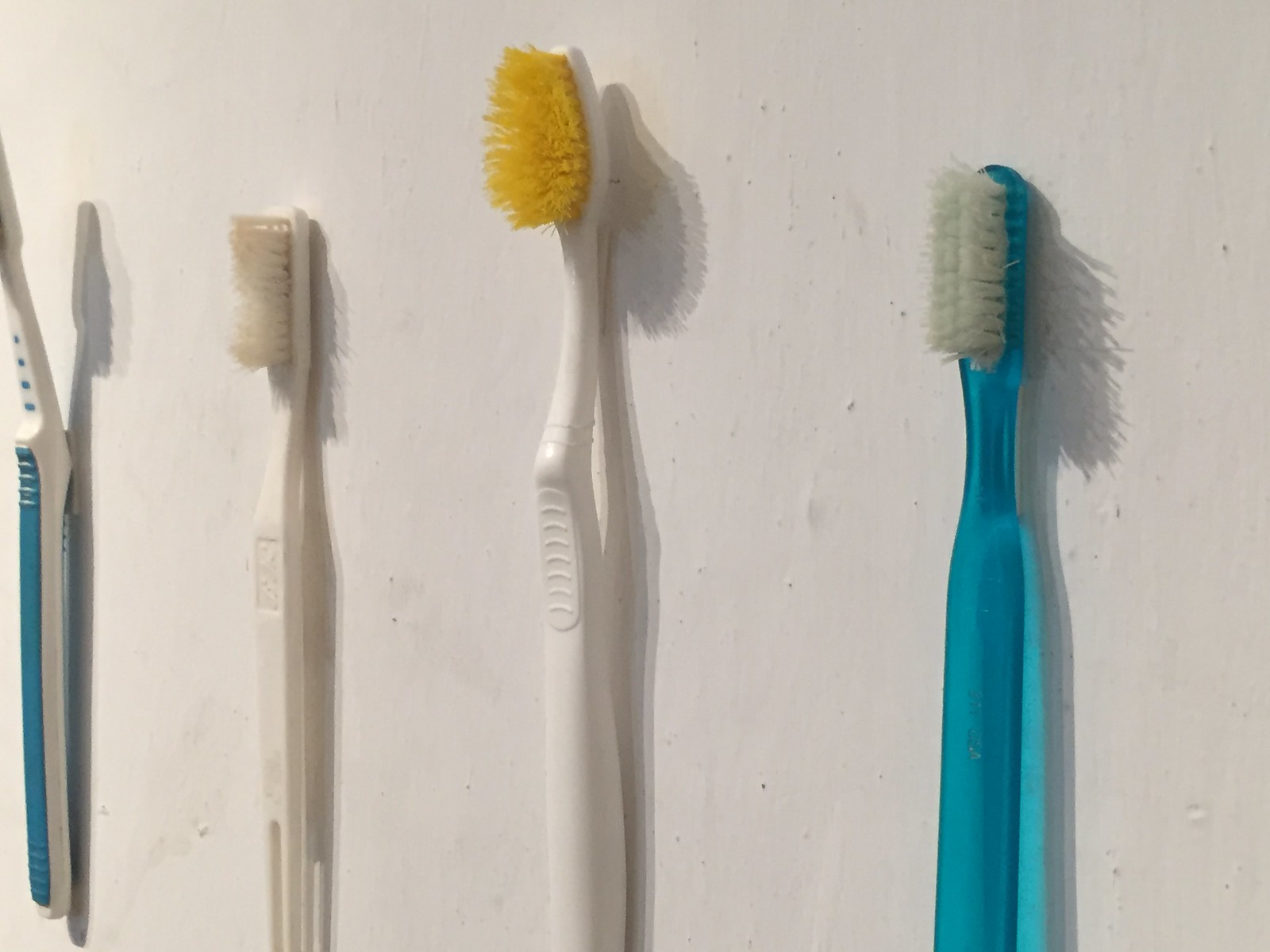This is a color photograph of four well-used toothbrushes lying horizontally on a white surface, but the image is rotated to make them appear as if they are vertically defying gravity against a wall. The toothbrushes are arranged from left to right. The first toothbrush on the left is white with blue grips, partially cropped so the bristles are not visible. It has a bent neck, possibly a Colgate. The second toothbrush is entirely white with off-white bristles and a thumb grip near the head, indicating heavy use. The third toothbrush is also white but notable for its yellow, pushed-in bristles, suggesting it is quite old. The fourth toothbrush, on the far right, is translucent blue with an oblong head and white bristles that are also well-worn. The light source coming from the left casts shadows to the right, adding depth to the composition.